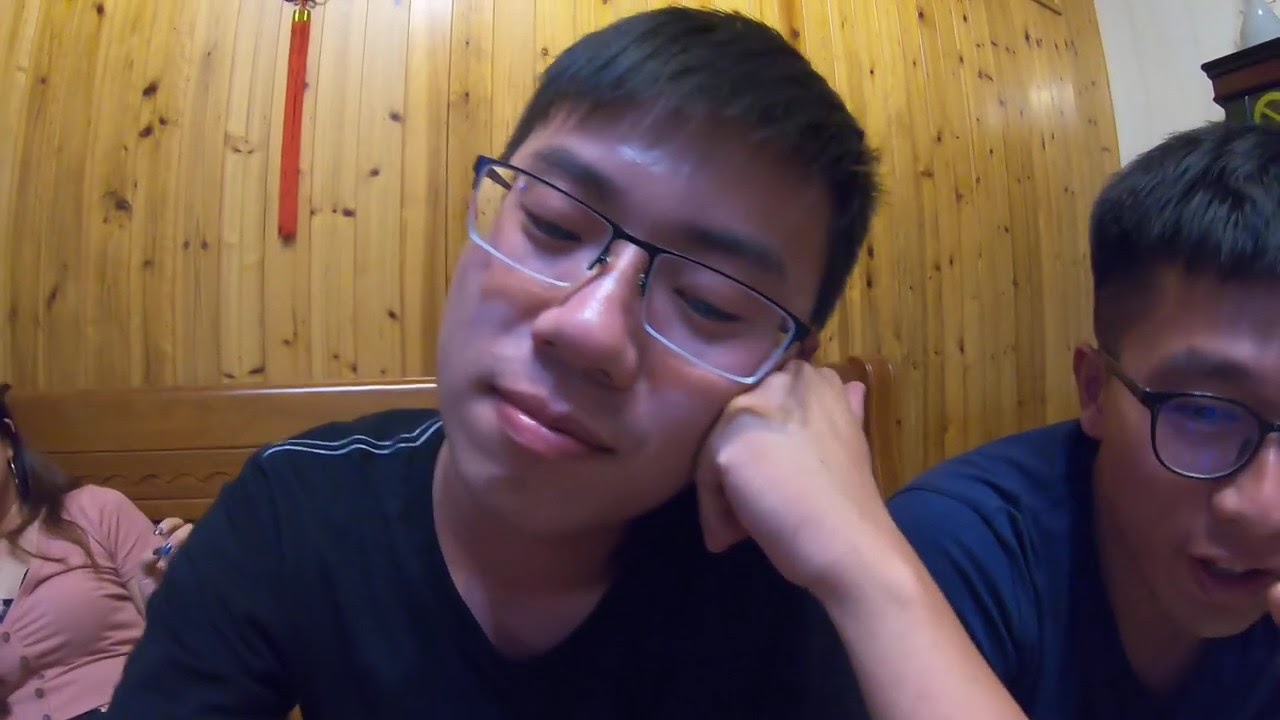In this close-up photograph, likely taken with a smartphone or webcam, the central focus is a young Asian man with short black hair and glasses, wearing a black t-shirt. He leans his face on his hand, appearing relaxed or slightly sleepy, with his eyes shut and a subtle smile. To the right of the central figure is another young Asian man, also in glasses and a blue shirt, with only half of his face visible. In the bottom left corner, a woman with dark brown hair and blue fingernails, dressed in a peach-colored top with buttons, leans partially out of frame, showing just her ear and shoulder. The setting appears to be an indoor space, possibly a den, characterized by wooden paneling on the wall and a brown wooden bench behind the young men. The overall lighting is decent, and there is a tassel from a graduation cap hanging on the wall behind them.